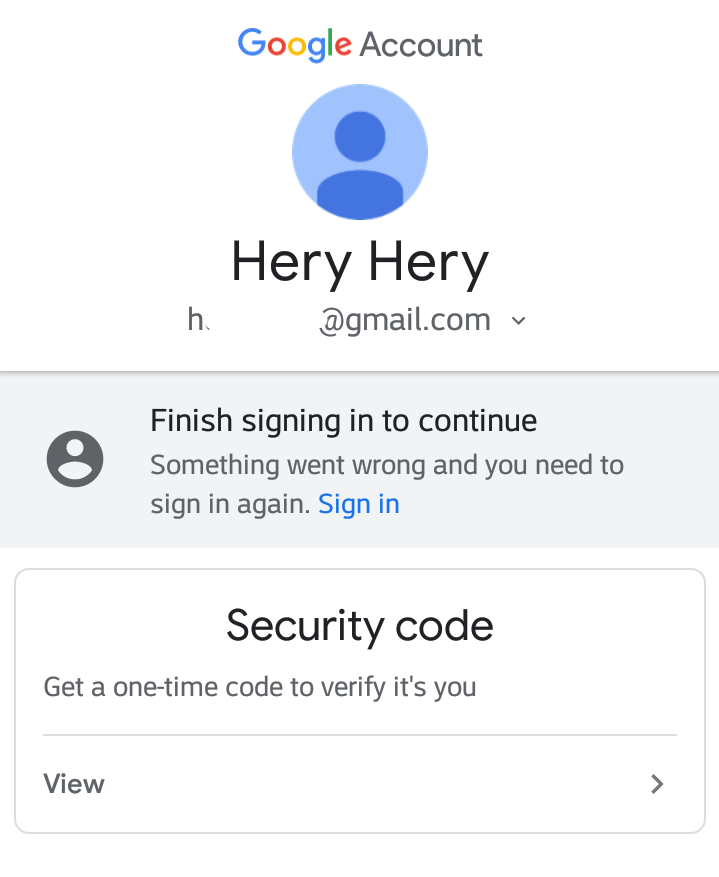This image is a detailed screenshot of a Google account sign-in verification page. At the top, the familiar "Google" logo is displayed in its signature rainbow colors, accompanied by the word "Account." Below this header is a blue circle icon featuring a silhouette of a person, indicating the user's profile. The user's name, "Harry," is repeated twice, followed by the phonetic spelling "H-E-R-Y, H-E-R-Y," and the partially obscured email address, which starts with "h" and ends with "gmail.com."

Beneath the profile information, a gray banner reads, "Finish signing in to continue. Something went wrong and you need to sign in again," accompanied by a clickable blue "Sign in" button. Following this, there is a text box labeled "Security Code," with a prompt underneath instructing users to "Get a one-time code to verify it's you." A thin line divider separates this section from a dropdown menu, indicated by the word "View" alongside a small arrow.

The screen is clearly designed for users who need to verify their identity before accessing their Google account, prompting them to obtain and enter a security code to proceed.